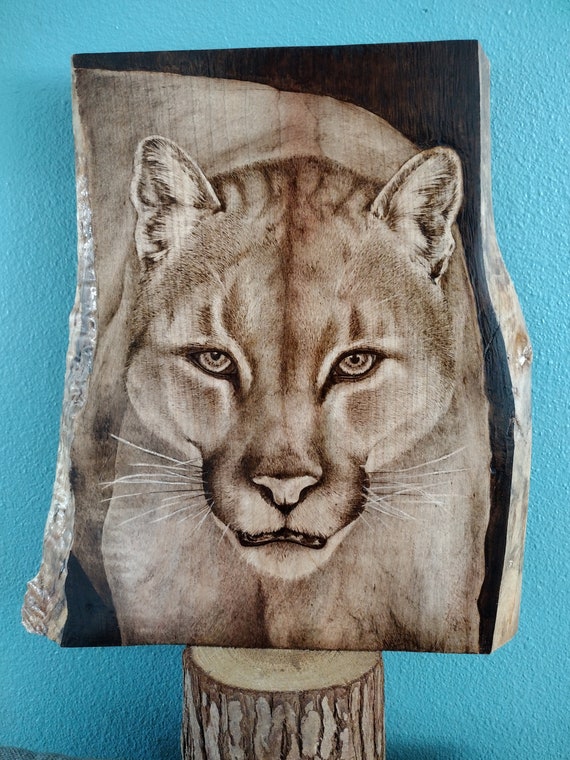The photograph captures an intricately detailed artwork of a cougar etched into a thick, tall slab of wood mounted on an elevated tree trunk stump. The wood slab, which features natural, rounded edges and a raw, textured appearance, showcases a remarkable image of a mountain lion. The cougar's face, meticulously burnt into the wood, displays lifelike features including faint head stripes, light tannish fur, black whiskers, and vivid eyes with black pupils surrounded by a brownish hue. The creature's nose appears lighter, contrasting against the darker brown shading around its forehead and nose, and its slightly open mouth reveals black lips and the hint of teeth. The background of the etched wood is stained a very dark brown, accentuating the wood grain. This entire artwork is positioned against a textured sheetrock wall painted in a turquoise or aqua green, enhancing the natural earthy aesthetics of the piece. The stand, made from a cut piece of tree trunk, has a scaly bark that adds to the rustic charm of the scene.